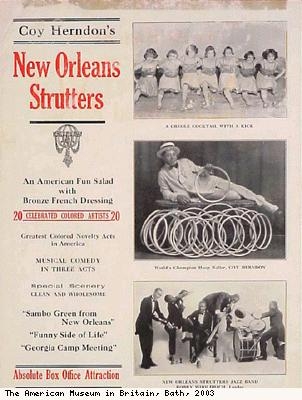The image is an advertisement for a live show, likely from the 1920s to 1940s, promoting "Coy Herndon's New Orleans Strutters." The text on the left, in black and red, highlights the show as "an American Fun Salad with Bronze French Dressing," indicating a musical comedy performance. The advertisement also emphasizes that it is an "Absolute Box Office Attraction" and notes its association with the American Museum in Britain, located in Bath, in 2003. On the right side, there are three black-and-white photographs: the top shows children dancing in white skirts, the middle features a man in a white suit and top hat lying on a stack of rings,  suggestive of a circus act, and the bottom illustrates a jazz band with drums, playing live music. The entire layout suggests a vibrant, multi-act show blending dance, circus performance, and jazz music from New Orleans.